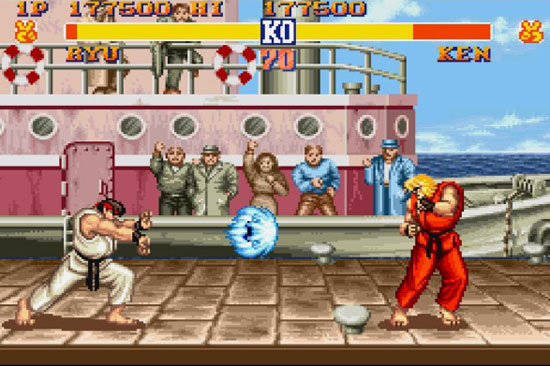The image depicts a classic fighting video game scene set on a tiled or paved floor resembling a rock-type pier, with a boat and cheering spectators in the background against a backdrop of water and blue skies. On the left stands a male fighter with brown hair in a white karate gi and black belt, his hands thrust forward as if launching a blue energy blast. On the right, his opponent, a muscular, blonde-haired male donning a red karate gi and black belt, braces himself in a defensive stance. The game characters are barefoot, and the red-clad fighter wears wristbands. Between the fighters, the blue energy blast is prominently visible, indicating an imminent strike.

The spectators on the boat are somewhat crudely drawn and include a bald man in a green shirt, a man in a gray trench coat and hat, a woman in a brown dress with one arm raised, a blue-shirted man beside her, and another male in a lighter blue coat and hat with one arm lifted in a cheering motion. Above, a scoreboard displays game statistics: "1P 17750 HI 17750," with red and yellow lifeline bars that include the characters' names, "RIU" (commonly "Ryu") and "Ken," along with a "KO" indicator. The scoreboard also features peace signs, signifying rounds won by each fighter. This lively scene captures the tension and intensity of a match between two iconic video game characters.